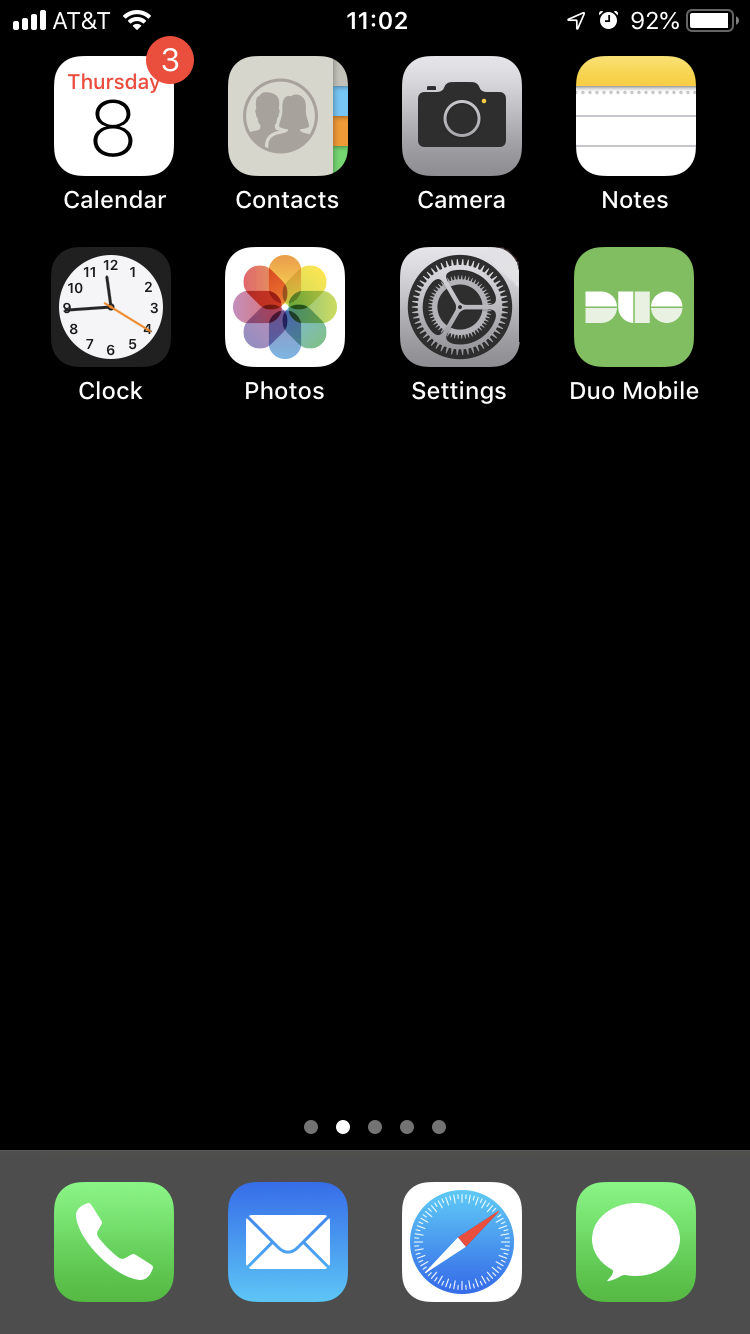This screenshot captures the app area of an iPhone in dark mode. At the top, the status bar showcases essential information on a black background. From left to right, it displays full signal strength with four bars, the AT&T network name, and a fully connected Wi-Fi icon. Centrally positioned, the time reads 11:02. On the right side, there are icons for location services, an active alarm clock, the battery percentage at 92%, and a horizontally oriented battery icon.

Below the status bar, two rows of four app icons are visible. In the upper row, the first icon is the Calendar app, indicating "Thursday 8" with a notification badge showing the number three in a red circle. Following this, the icons for Contacts, Camera, Notes, and Clock are aligned. The second row features icons for Photos, Settings, Duo Mobile, and an additional Clock app icon.

The remainder of the screen is mostly empty, highlighting the stark black background which emphasizes five small navigation dots at the bottom, indicating multiple home screens. The second dot is highlighted, signifying that the user is on the second screen.

At the very bottom of the screenshot, the iPhone's dock is shown against a dark gray background. The dock contains four essential apps: the Phone app, Mail app, Safari browser, and the Messages app, which is easily recognizable as a green icon with a white chat bubble.